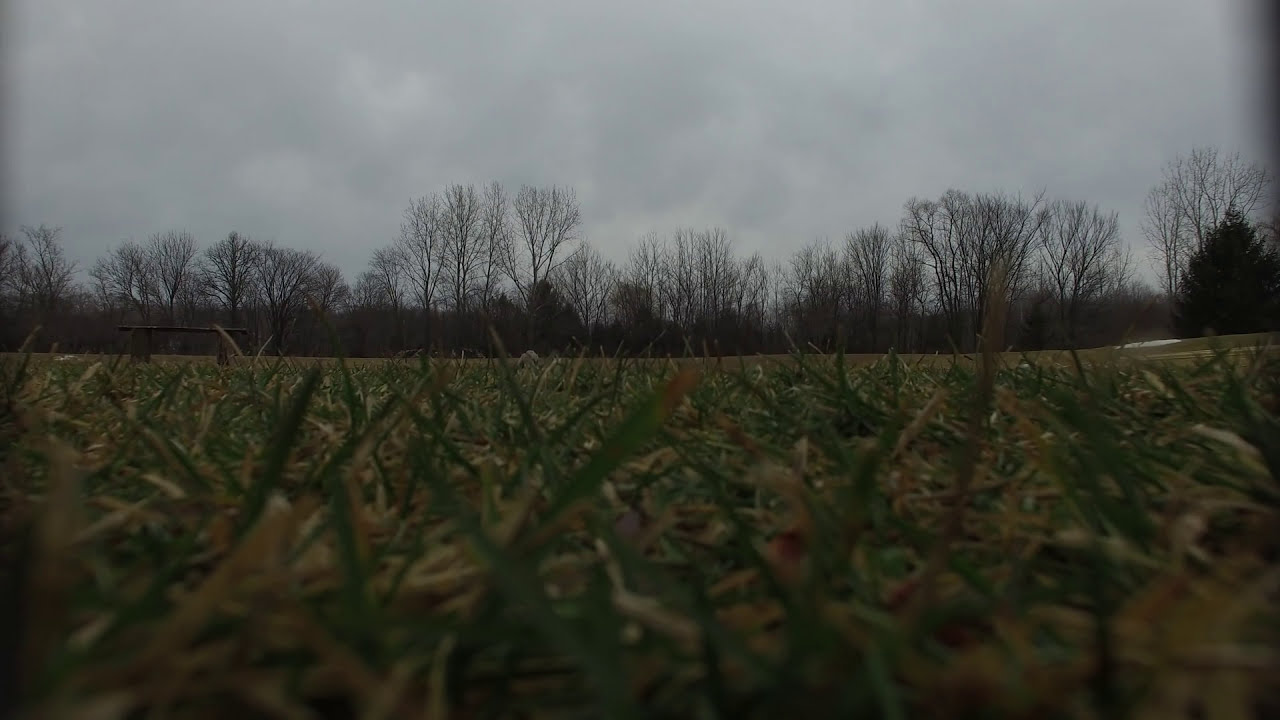This photograph captures a close-up view of a grassy area, taken from a very low angle, almost as if lying on the ground. In the foreground, some blades of grass appear blurred due to their proximity to the camera lens, creating a vivid sense of depth. The grass is a mix of green and tan hues, indicating that some blades are alive while others are dying or dead. 

Behind the grass, the middle ground reveals more greenery and a possible small structure, likely a wooden table or bench, located on the left-hand side. The background features a row of mostly leafless deciduous trees extending across the frame, hinting at a late winter or early winter timeframe. Interspersed among the bare trees are a few evergreen coniferous trees, including a noticeable, triangle-topped fir tree on the right side. 

The upper half of the image is dominated by a gray, overcast sky that appears heavy with clouds, contributing to the overall dark, dank atmosphere of the scene. The combination of greens, browns, and grays paints a muted, somber picture, devoid of sunlight and vibrant colors.